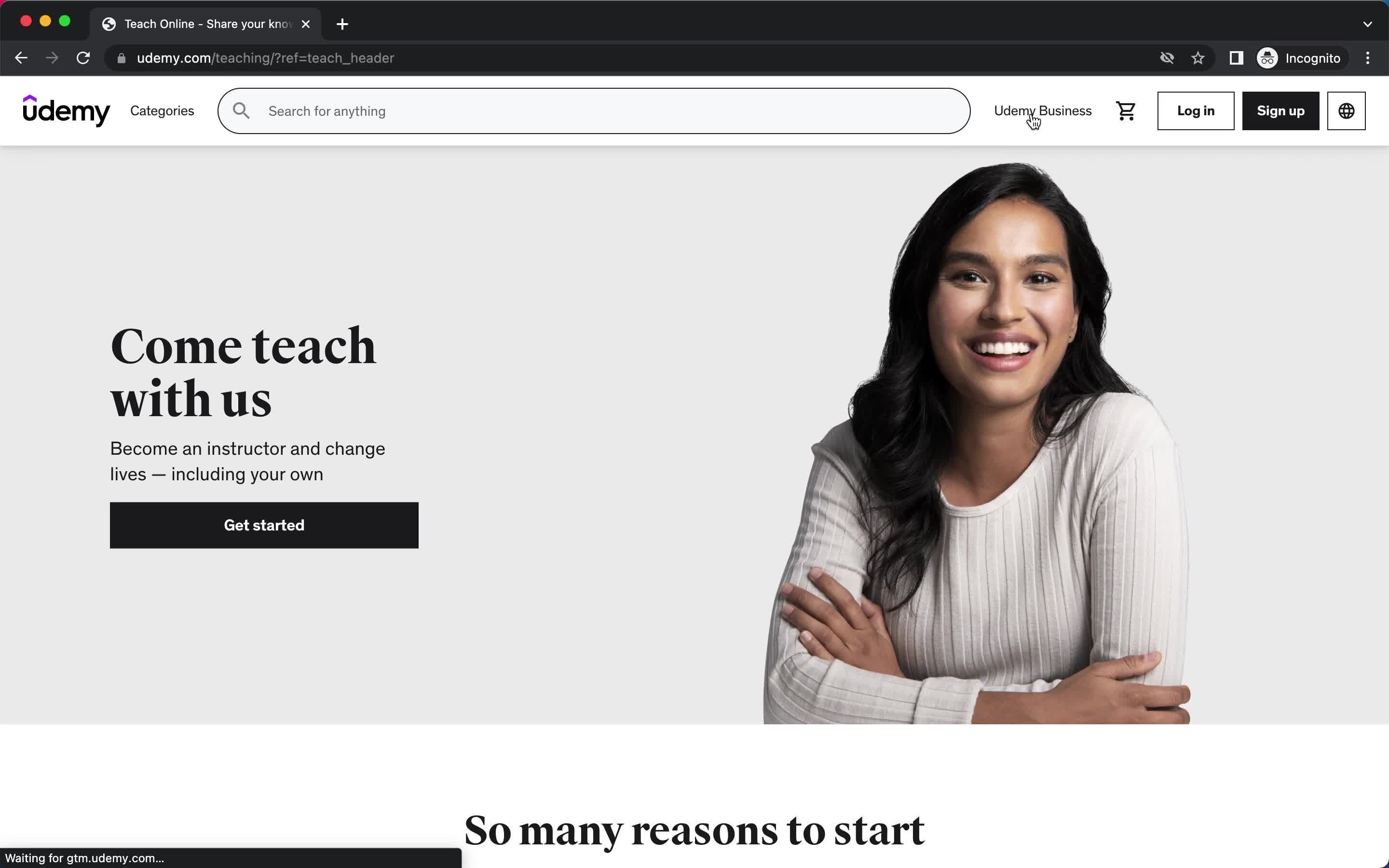Screenshot of the Udemy.com homepage in incognito mode. The header of the website is black, prominently featuring the Udemy logo, which has a purple tilde over the "U" and the rest of the text in black. The main section of the page showcases a photo of a woman with black hair, wearing a white long-sleeve shirt with horizontal stripes. She is smiling and crossing her arms over her chest. The text adjacent to her image reads, "Come teach with us, become an instructor, and change lives, including your own." The browser window shows three small dots in the upper left corner, colored red, yellow, and green, indicating the user is in incognito mode.